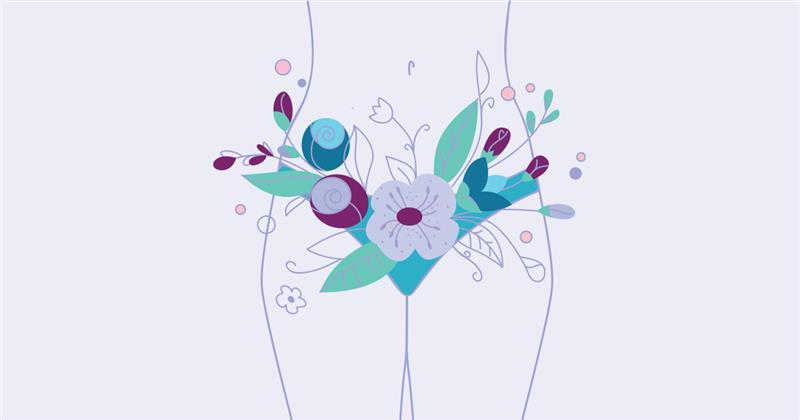The image depicts a detailed artwork with a white background featuring an outlined, stylized female body from just above the waist to slightly below the knees. The figure appears to be adorned with underwear, which can be imagined as a blue-green hue, intricately interwoven with a vibrant array of flowers and leaves. The central floral element is a whitish flower with a maroon center, surrounded by darker blue and green petals, strategically placed to cover the crotch area. Additional floral details include smaller maroon and blue tulip-shaped flowers, some rounded buds resembling roses, and delicate stems and leaves that extend outward from the main floral arrangement. On the left side, there's a prominent dark blue circular plant, complemented by smaller green and pink accents. The overall composition suggests a harmonious blend of floral and anatomical artistry, emphasizing the natural beauty and complexity of both.